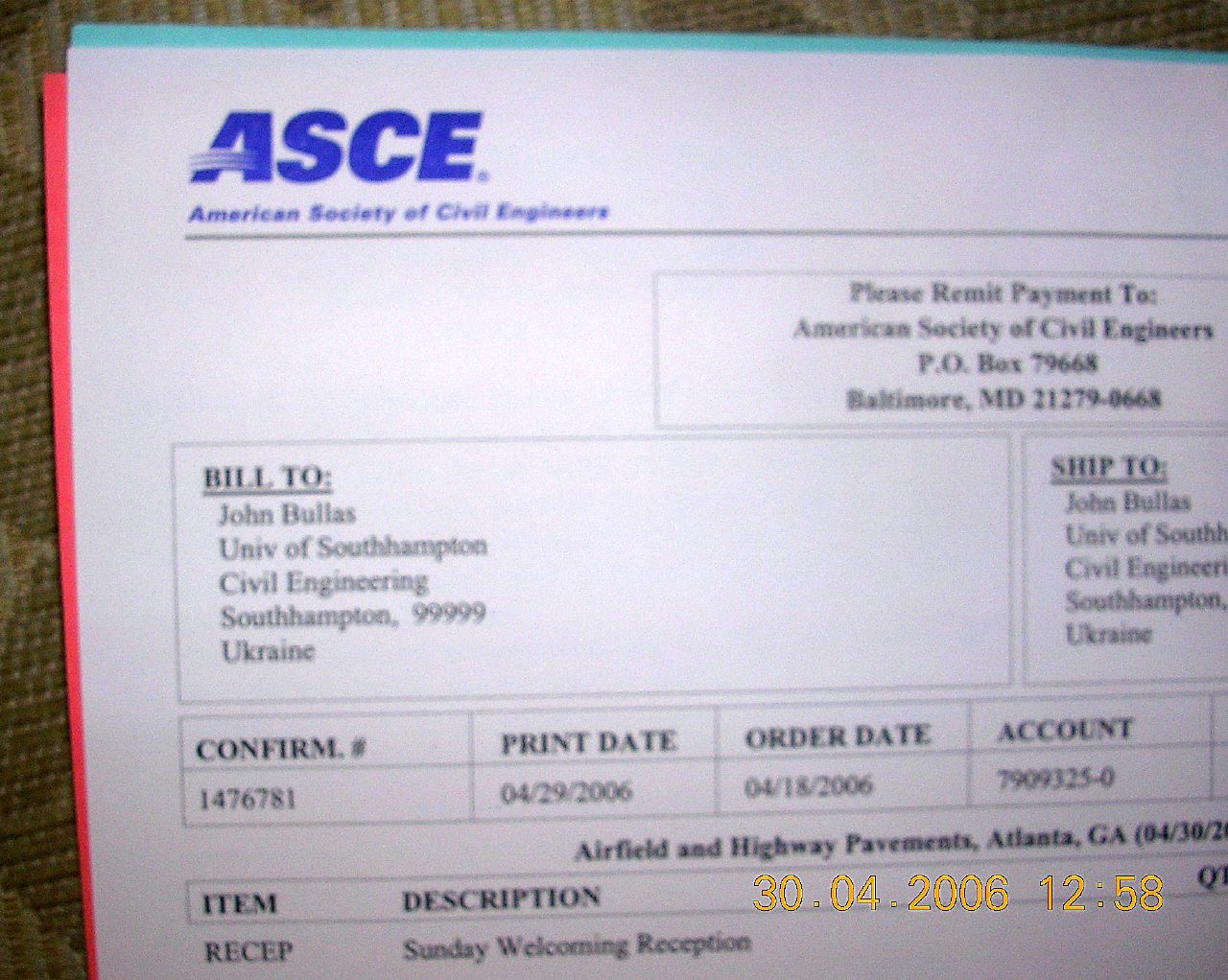The photograph features a bill on a company's letterhead placed on a brown wooden desk. The bill prominently displays the letters "A-S-C-E" in bold blue capital letters at the top, representing the American Society of Civil Engineers. Below this, in a black line, it reads "American Society of Civil Engineers," followed by a rectangle enclosed with a black border that instructs "Please remit payment to American Society of Civil Engineers, PO Box 79668, Baltimore, Maryland, 21279-0668." The bill is addressed to "John Bullis, University of Southampton Civil Engineering, Southampton 99999, Ukraine," under both "Bill to" and "Ship to" sections. Additional details such as the confirmation number, print date, and order date are mentioned along with a timestamp at the bottom right indicating "30.04.2006 12:58" in yellow. The top half of the page features a turquoise color, while the left-hand margin is highlighted in red.